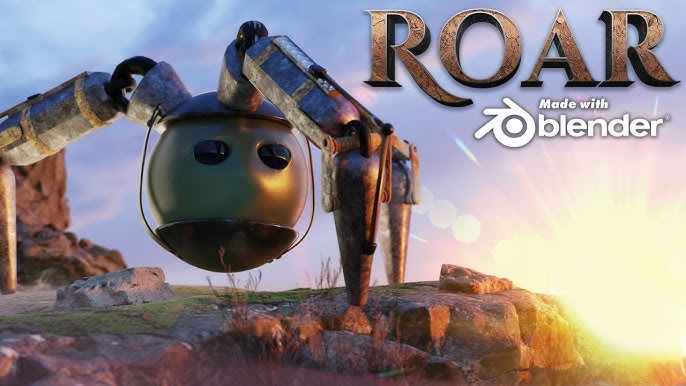The image features a robotic entity prominently positioned in a rugged, rocky terrain, reminiscent of a cliffside environment. The robot itself is distinctly spherical with a smooth, polished surface, and prominently displays two black circles, likely suggestive of eyes. Uniquely, it stands on three slender, angular legs that originate from the top of its body, closely resembling the legs of a spider, tapering sharply at the points where they touch the ground.

In the immediate vicinity of the robot, patches of greenery and small tufts of grass dot the rocky soil, adding a touch of life to the stark landscape. The background unveils a clear, blue sky, accentuating the scene's natural beauty.

Adding an artistic touch to the image, the phrase "ROAR" is boldly presented in three-dimensional brown letters in the top-right corner. Directly beneath this label, the words "Made With Blender" are inscribed in white, accompanied by the Blender logo, signifying the software used to create this artwork.

The scene is further dramatized by a vivid sunrise or sunset in the bottom-right corner, with radiant sunbeams extending outward. The sky transitions from a bright, sunny yellow to an enchanting gradient of pinkish-orange hues, providing a warm and visually appealing contrast to the mechanical figure at the center of the image.